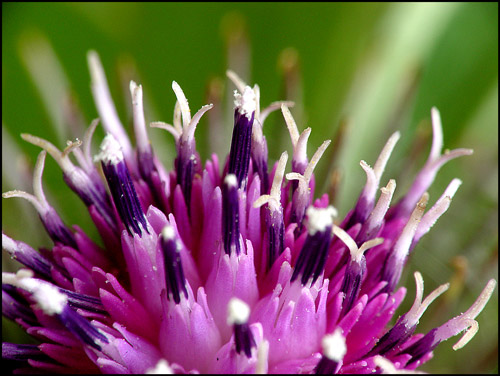The image is a close-up, macro photograph of an unusual and striking flower, showcasing the intricate details of its pink, purple, and white hues. The flower appears to be partially closed, with various small tentacle-like protrusions and tiny specks of pollen visible, possibly on its stamens. The background is an abstract, watercolor-like blur of green shades, resembling grass or other plants, enhancing the focus on the flower's vivid colors. Although the petals are out of shot, the center of the flower dominates the image, drawing attention to its detailed textures and vibrant palette. The overall style is naturalistic, emphasizing the delicate and captivating beauty of the flower against a softly muted backdrop.